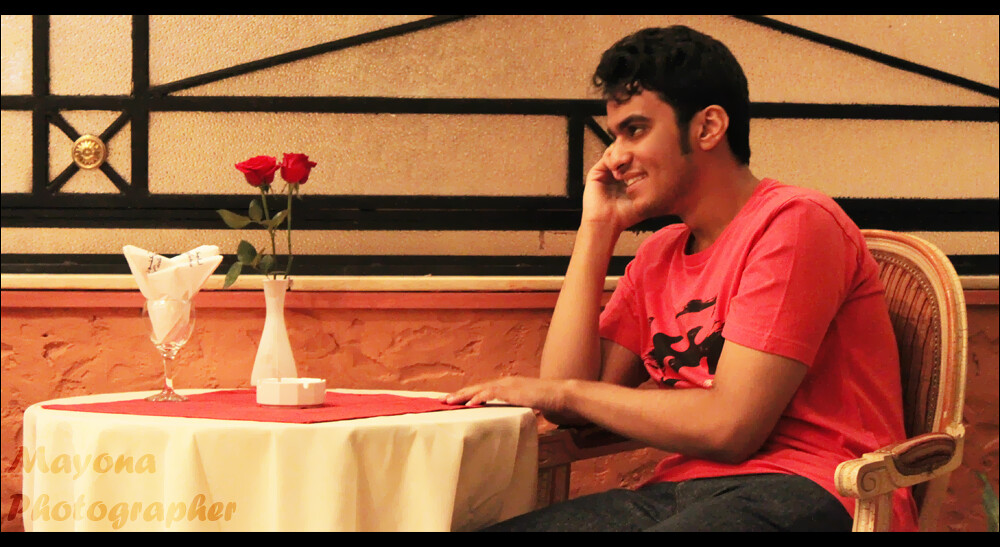A young man, dressed in a rose-colored t-shirt with a black design and wearing blue jeans, is seated alone at a small table in an outdoor cafe. His dark hair and long sideburns frame his smiling face as he talks into his cell phone, with his right hand up near his ear. The table in front of him is set with a white vase holding two red roses and a champagne glass with a folded white napkin. Additionally, a white ceramic ashtray is placed on the table. He sits in a cane chair with wooden arms. Behind him, the wall features a goldish square pattern on the upper half and a salmon-colored stucco texture on the bottom half, adding warmth to the overall ambiance.